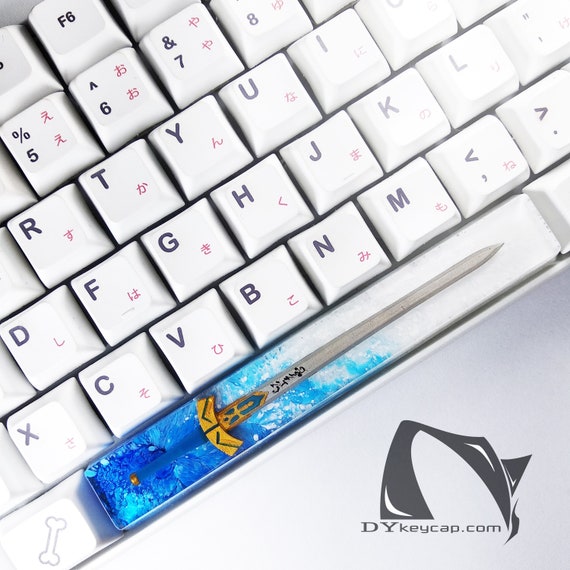This image, predominantly square in shape, showcases an up-close and detailed portion of a keyboard. The keyboard, which appears at an angle, features a white base with gray keys, black lettering, and small red Chinese or Japanese symbols beneath the characters. Key sections visible include F6, the numbers 5 through 8, the letters R, T, Y, U, I, D, F, G, H, J, K, L, semicolon, and the lower row letters X, C, V, B, M, comma, and period. The standout feature is the spacebar, which transitions from blue to gray and is adorned with a long, blue and gold sword graphic, accompanied by some black writing in Japanese or Chinese. On the right corner of the keyboard, there is a dog bone symbol on the alternate key and a logo that reads "dykeycap.com" with an abstract design above it. The entire keyboard is set against a faded gray background, enhancing the visibility and detail of the keys and symbols.